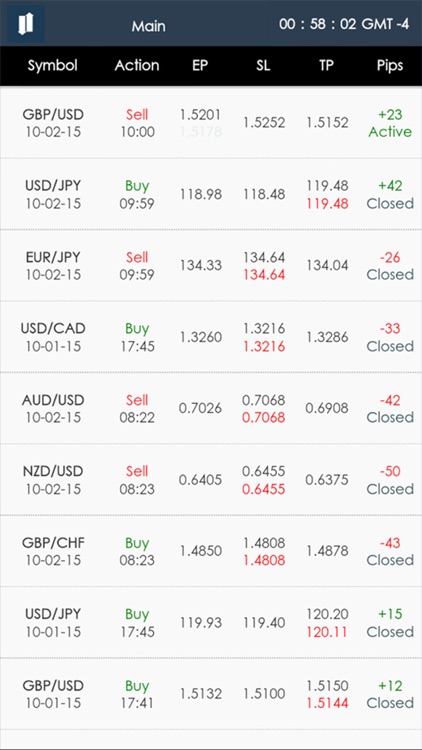A detailed description of the image shows a screen capture, likely taken on a smartphone, depicting a stock market watch or trading application. At the top of the screen, there is a gray bar with the text "Main" in white and a timestamp reading "00:58:02 GMT -4." Directly beneath this is a black bar labeling six columns from left to right as follows: Symbol, Action, EP, SL, TP, and PIPS.

Under the "Symbol" column, the listed currencies being monitored are:
- GBP/USD
- USD/JPY
- EUR/JPY
- USD/CAD
- AUD/USD
- NZD/USD
- GBP/CHF
- USD/JPY
- GBP/USD

In the adjacent "Action" column, buy and sell options are indicated, with "Buy" entries highlighted in green and "Sell" entries highlighted in red. Further to the right, the screen displays the trading status, where active trading sessions are marked in green, and closed sessions are marked in red.